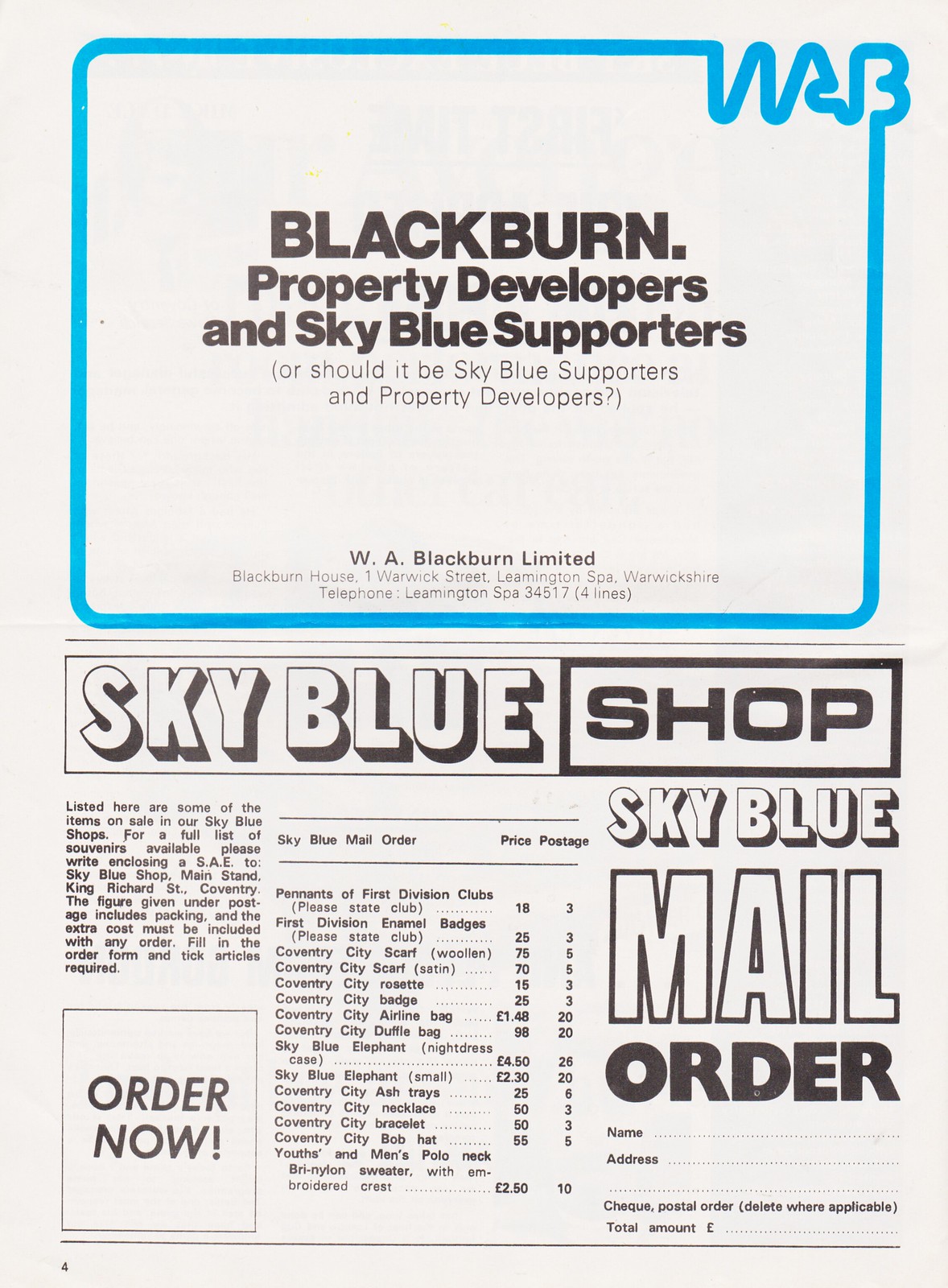The image depicts a page from a magazine that primarily features advertisements for the same business, likely related to Blackburn Property Developers and the Sky Blue supporters. The top half showcases a blue-bordered rectangle filled with white background and black text, stating: "Blackburn Property Developers and Sky-Blue Supporters" or "Sky-Blue Supporters and Property Developers." It also lists the business address as WA Blackburn Limited, Blackburn House, 1 Warwick Street, Leamington Spa, Warwickshire with the telephone number Leamington Spa 345174 lines.

The bottom half of the page focuses on a mail order advertisement for the "Sky-Blue Shop." It mentions various items available, with a specific note in small black letters indicating, "Listed here are some of the items on sale in our Sky-Blue Shops. For a full list of souvenirs available, please write enclosing a SAE to Sky-Blue Shop Main Stand, King Richard Street." It includes details on the ordering process, emphasizing that the given postage figure includes packing and the extra cost must be added to any order. The bottom left corner features an "Order Now" prompt, along with spaces for name, address, and check details, as well as instructions to fill in the order form and tick off required articles.